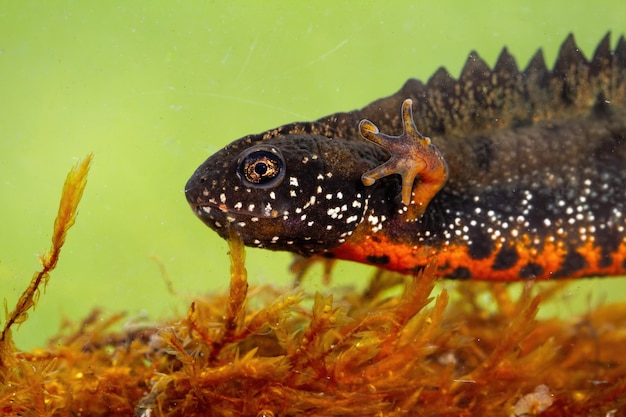The image depicts a close-up of an iguana-like creature, possibly underwater or in an aquarium, with no text present. Dominated by a palette of lime green and yellowish-orange, the picture also includes contrasting blacks and browns. The creature features a scaly black and brown body with an orange underbelly speckled in black. Its elongated body extends from the middle right toward the center, with its head pointing to the left. Its back hosts a series of small spines that run down the spine, ending just before the image cuts off at the creature's midsection. The limbs visible in the frame are webbed, enhancing the aquatic ambiance. The background features lime green hues and brownish grasses or plant life, embellished with hints of mercury-like reflective qualities. The creature's gold-colored eyes offer a no-nonsense, almost bored expression, while its hidden mouth leaves its true demeanor a mystery.